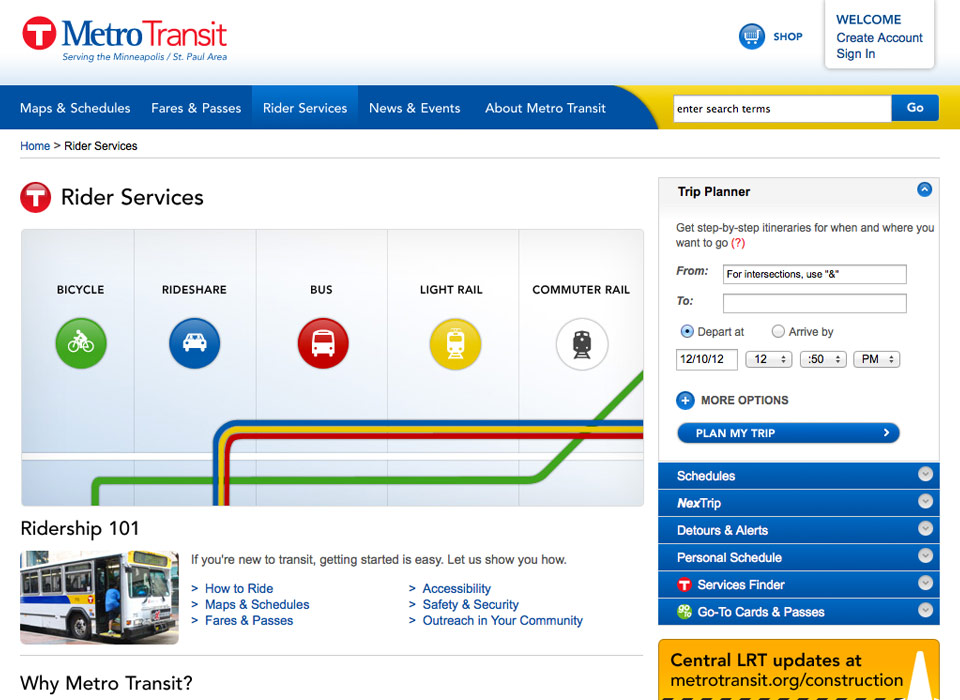This is a screenshot from the Metro Transit webpage, with a clean and organized layout against a white background. In the upper left corner, there is a prominent red circle with a white "T" at its center, followed by "Metro" in blue text and "Transit" in red text. Just below this logo, there is a tagline in blue text that reads, "Serving the Minneapolis-St. Paul Area."

On the right-hand side of the page, there is a round blue button featuring a shopping cart icon, accompanied by the word "Shop." Further to the right, the options "Welcome," "Create Account," and "Sign In" are displayed.

Directly beneath the header, a blue navigation bar spans the width of the page, featuring white text with categories such as "Maps and Schedules," "Fares and Passes," "Rider Services," "News and Events," and "About Metro Transit." A search function is incorporated within a yellow rectangle that includes a white text box labeled "Enter Search Terms" and a blue "Go" button.

Following this, a breadcrumb navigation shows "Home" > "Rider Services." Below this, the familiar Metro Transit "T" emblem appears again next to the "Rider Services" section, which includes links to "Bicycle," "Rideshare," "Bus," "Light Rail," and "Commuter Rail."

To the far right, a vertical rectangle features a comprehensive trip planner tool, inviting users to "Get step-by-step itineraries for when and where you want to go." The tool includes text boxes for "From" and "To" locations, options to "Depart at" a specific time or "Arrive by" a specific time and date, followed by more options for customization. Below these fields, buttons and links are provided for "Plan My Trip," "Schedules," "Next Trip," "Detours and Alerts," "Personal Schedule," "Services Finder," and "Go-To Cards and Passes."